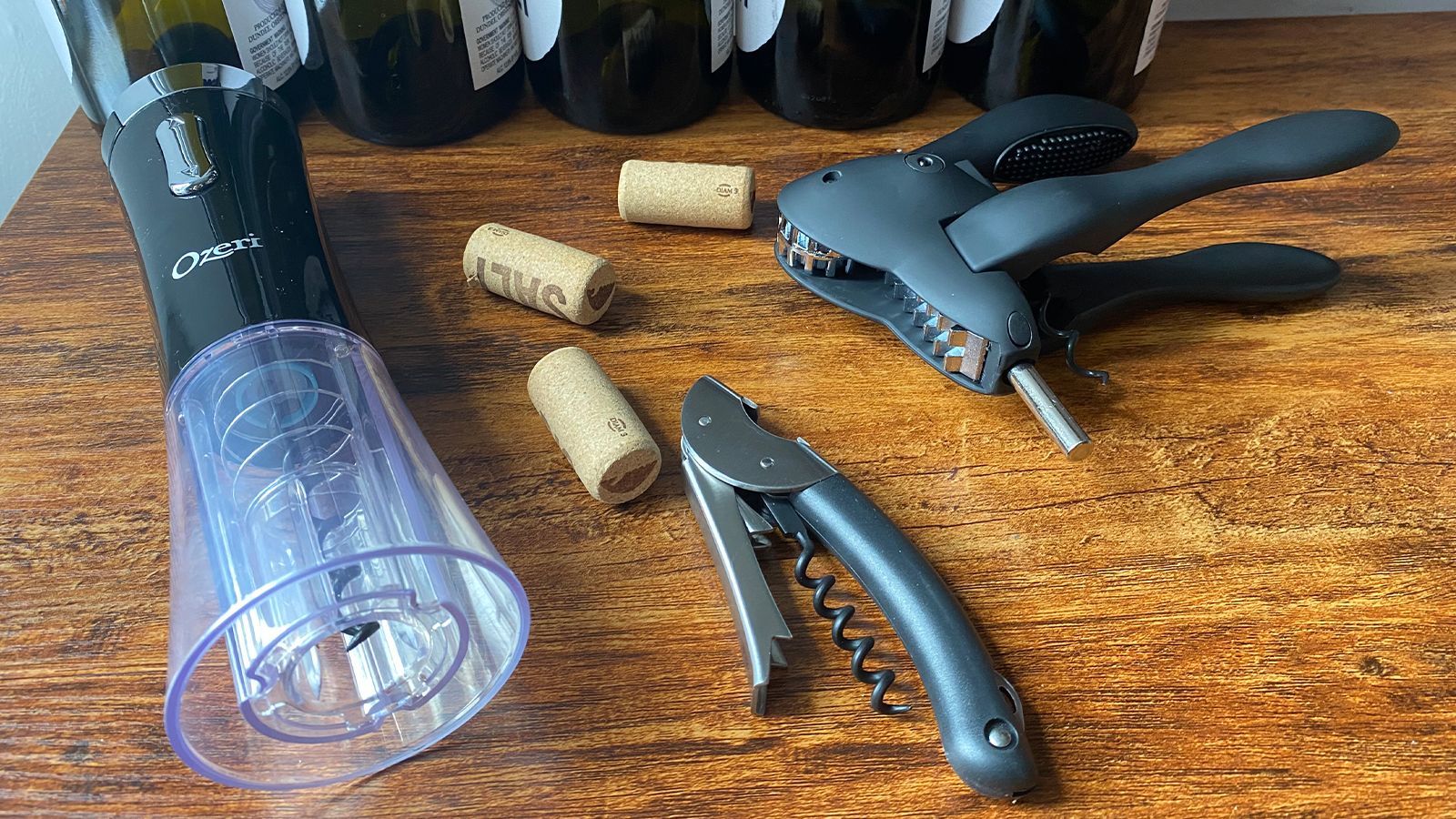The image showcases a detailed array of wine opening tools displayed on a polished, dark wooden table, possibly walnut, in a wine bar or winery. Prominently featured are three different styles of wine bottle cork removers. On the far left is a sophisticated, automated cork remover, encased in clear plastic at the bottom with a black top and a button on it, designed to seamlessly extract the cork. The image also highlights three wine corks arranged in the center, indicative of recent use. To the right of these corks are two manual corkscrews: one is a traditional, spiral-designed pigtail corkscrew, and the other is a more advanced manual cork remover resembling a pistol grip for better leverage. Behind these tools, five wine bottles stand in various states of emptiness, with the far-left bottle appearing empty. The entire setup exudes a clean, professional ambiance, enhanced by the lacquered wood grain table that serves as an elegant backdrop. One cork bears an inscrutable "salt" marking, adding a touch of mystery to the display.